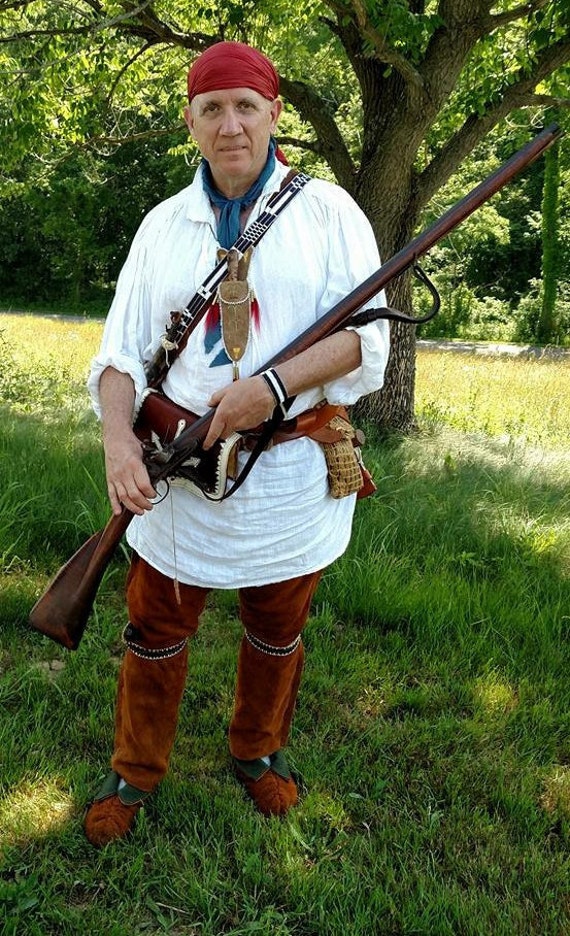In this daytime outdoor photograph, you see a man standing on lush green grass with trees in the background and the sun shining overhead. He is dressed in a vibrant costume featuring a red bandana on his head and a long white shirt that almost reaches his knees, adorned with a red belt and fanny pack with white accents. The man also wears a blue scarf and a gold medal that dangles from the belt to the fanny pack. His lower attire consists of distinctive red pants and red boots, which are embellished with green around the feet and silver around the knees. He holds a long rifle, a musket, across his body with both hands. A white bracelet with black ends is visible on one of his wrists. There is also a strap over his shoulder, hinting at something carried on his back that is not visible in the image. The man's attire and accouterments, including the rifle, suggest an old-fashioned or possibly Native American-inspired look. The background features a large tree with green leaves, enhancing the natural, backyard setting.